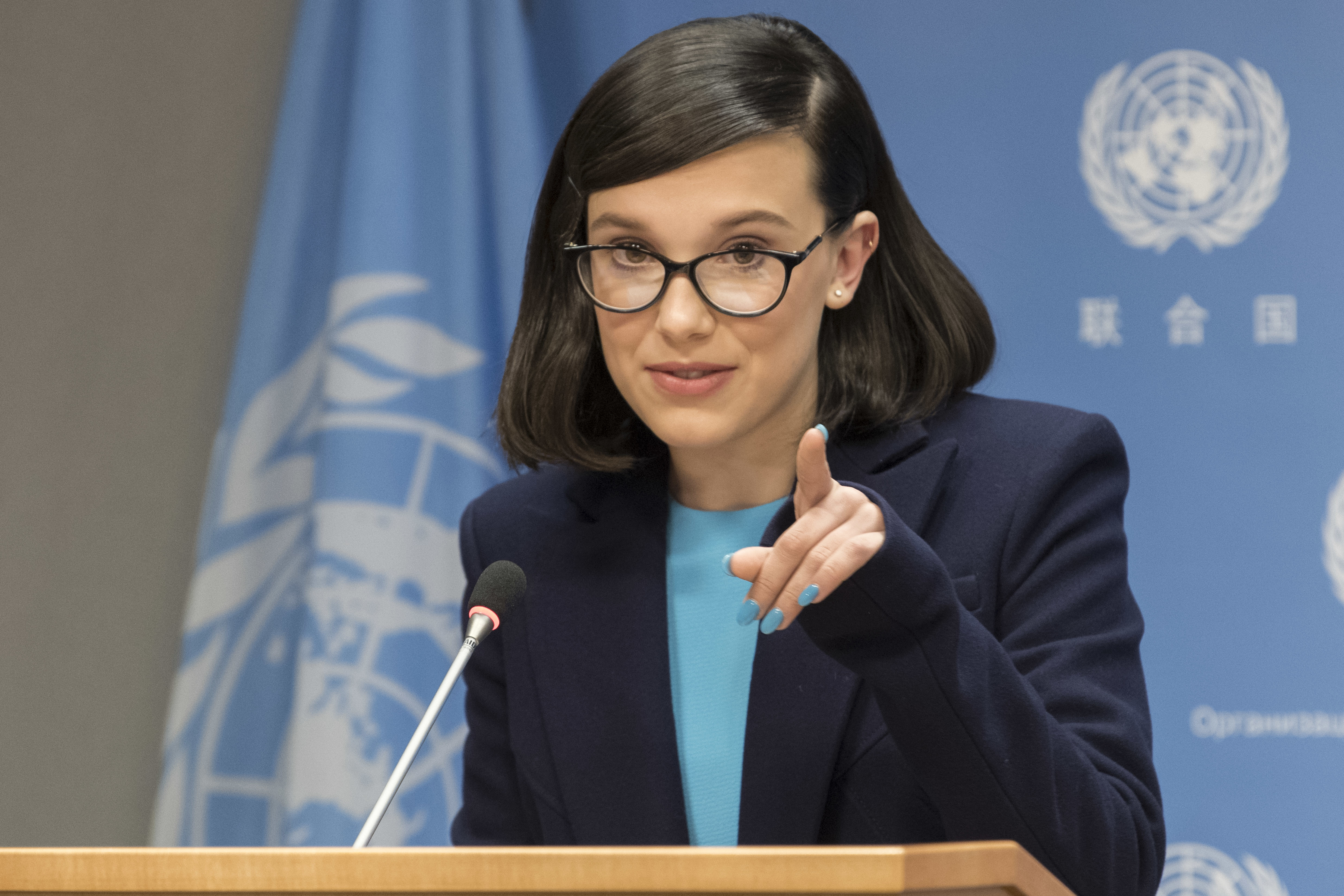A young Caucasian woman with light pale skin is standing at a podium made of light brown wood, speaking into a microphone that has a silver metal base with a black top. She wears a navy blue blazer over an aqua blue boatneck top, with her nails painted to match the top. Her dark black bob haircut extends just past her chin, and she sports dark-framed glasses, little pearl earrings, and a cartilage piercing. Behind her, there is a light blue backdrop and a flag, both featuring a white circular logo with leaves on either side and white characters, likely representing the United Nations, though they are out of focus. The woman appears to be gesturing with one hand, pointing, and looking almost directly at the camera.